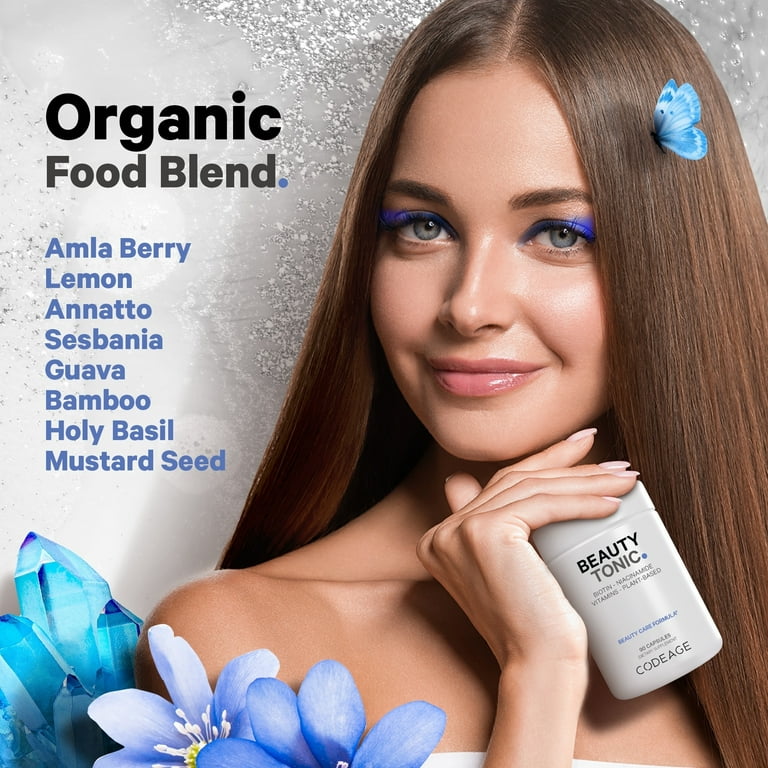The advertisement features a strikingly beautiful young woman with long, very straight brown hair adorned with a delicate butterfly clip and aqua blue flowers. Her flawless, slightly tan skin contrasts with her vivid blue eyeshadow, which complements her bright blue eyes and soft pink lipstick. She is positioned on the left-hand side of the square-shaped photo, taking up the majority of the image and giving a frontal view that includes her bare shoulders.

She is holding a bottle of Beauty Tonic from a company called Code Age (or possibly Kodige, NACRNAMD, as different captions suggest slight variations in naming). The bottle text highlights its plant-based composition, mentioning ingredients such as Amla Berry, Lemon, Annatto, Sesbania, Guava, Bamboo, Holy Basil, and Mustard Seed. The right-hand side features a slightly smudged, sparkly white background with black and bluish-purple text detailing the organic food blend ingredients. Additionally, blue flowers with a touch of yellow and turquoise petals are seen near her shoulder, which add to the overall aesthetic of the ad.